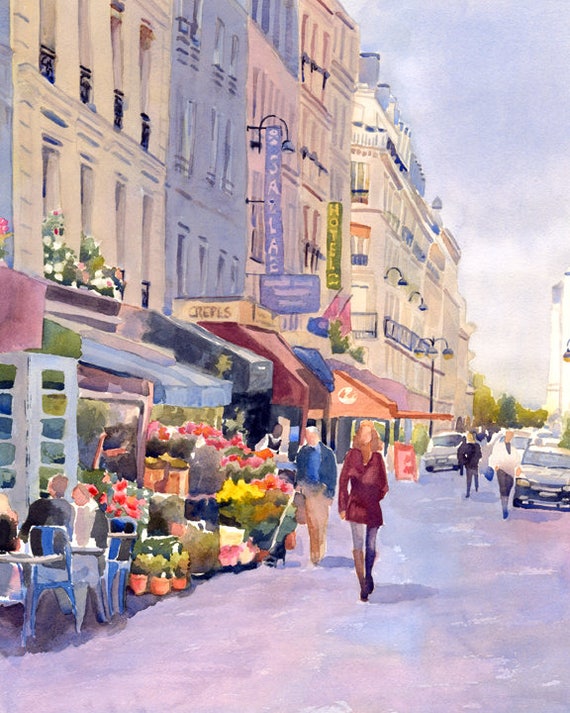This is a captivating watercolor painting by Rue Cler, showcasing the vibrant and bustling atmosphere of Parisian street life. The artwork beautifully captures the charm of French cafes in Paris, highlighting the multi-story buildings on the left adorned with intricate details and colorful awnings that shade the sidewalks below. Stalls brimming with fresh fruits and vegetables line the street, creating a lively market scene.

In the foreground, a woman dressed in a short coat or dress paired with knee-high boots stands gracefully, while a gentleman clad in a light blue jacket and khaki pants strolls by, adding a sense of movement and life to the painting. The artist’s use of watercolor paints adds a slightly exaggerated, impressionistic touch, making the scene both realistic and dreamlike.

Above the bustling sidewalks, elegant street lamps cast a warm glow, complementing the blue-gray sky overhead. Signs hang prominently in front of the buildings, guiding the way to the charming sidewalk cafe. Here, patrons sit in inviting chairs, conversing and savoring the ambiance. The cafe's open doors, framed by multi-pane windows, welcome visitors, and above these doors, flower boxes brimming with vibrant blooms add a touch of color and romance to the scene. This watercolor by Rue Cler encapsulates the essence and allure of Paris, offering a glimpse into the daily life and timeless beauty of the city.